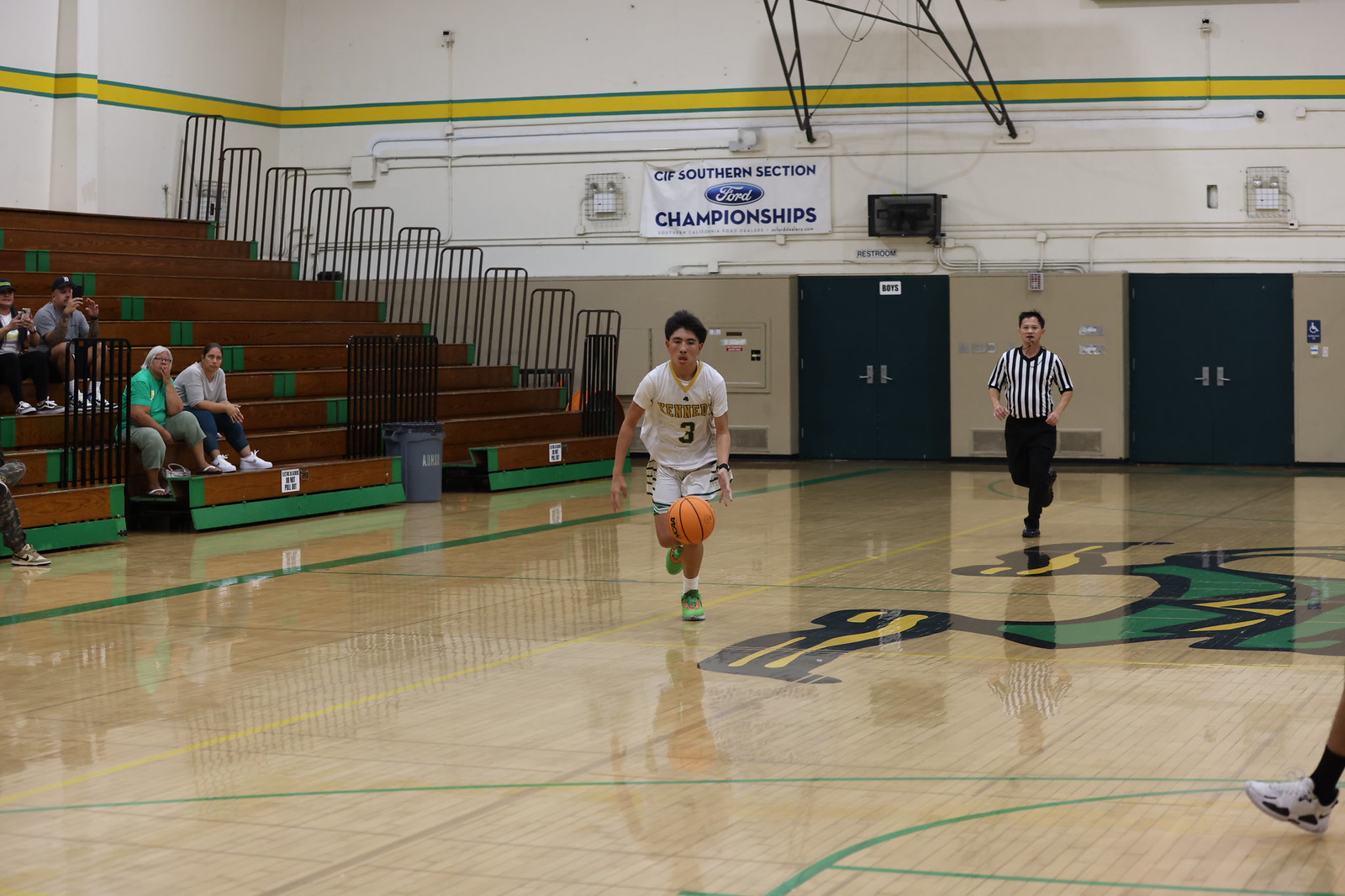In this detailed image set in a school gymnasium, a basketball player from Kennedy High School is captured in mid-dribble at center court. He wears a white jersey emblazoned with "Kennedy" in gold letters and a green number three, paired with white shorts and green sneakers. The floor is a polished light brown wood with green markings, and a prominent green and gold Fighting Irish emblem decorates the center.

Behind the player, a referee in a traditional pinstriped shirt and black pants can be seen running. The background features brown bleachers with green accents, sparsely populated with spectators. Above two black double doors at the back of the gym, a white banner reads "CIF Southern Section Championships" with the Ford auto logo prominently displayed. The scene captures the anticipation and energy of an ongoing or upcoming high school basketball game.